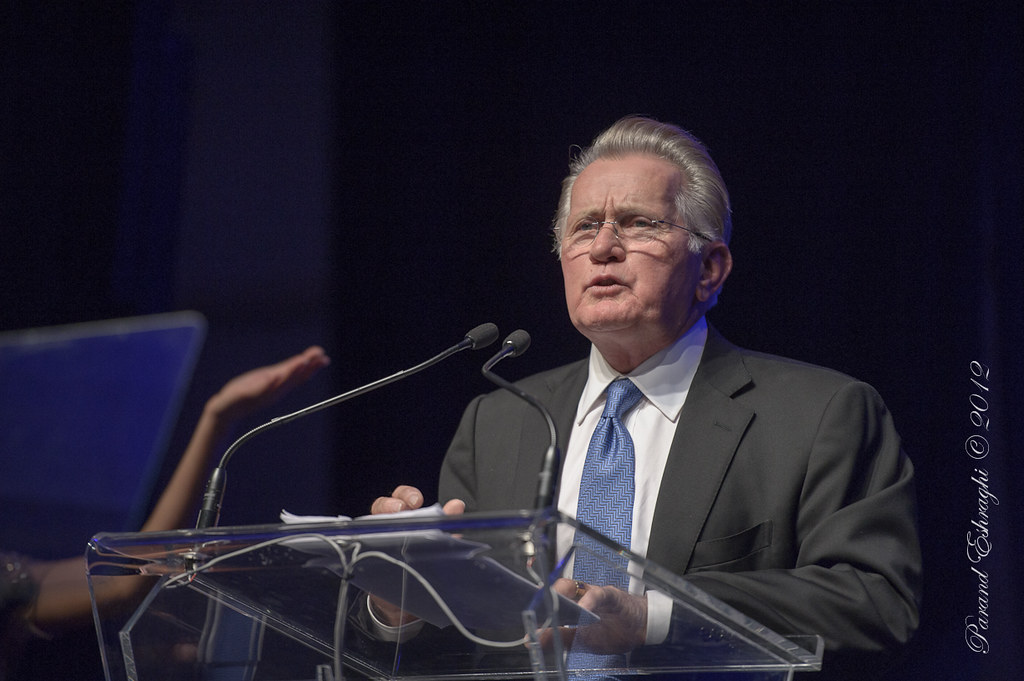In this image, we see a detailed setting with various elements. Predominantly, the background is black with hints of blue curtains. Centrally positioned in the image is an elderly man standing at a transparent glass podium, seemingly addressing a crowd. The podium features two microphones situated at his neck level. The man, who sports slicked-back gray hair, is dressed in a gray suit paired with a white button-down shirt and blue tie. He also wears thin circular glasses. His stance and expression suggest he is engaged in delivering a speech or sermon. To the left side of the image, an arm intrudes into the frame, bent at the elbow with the palm facing upward, indicating a gesture of praise or acknowledgment. While there's no immediate text visible on the primary image, the right-hand vertical side showcases some cursive writing: "Parand Eshraghi, copyright 2012." There is speculation that the speaker might be Billy Graham, given the context and setup. Overall, the scene is an indoor environment set up for a formal address or religious event.